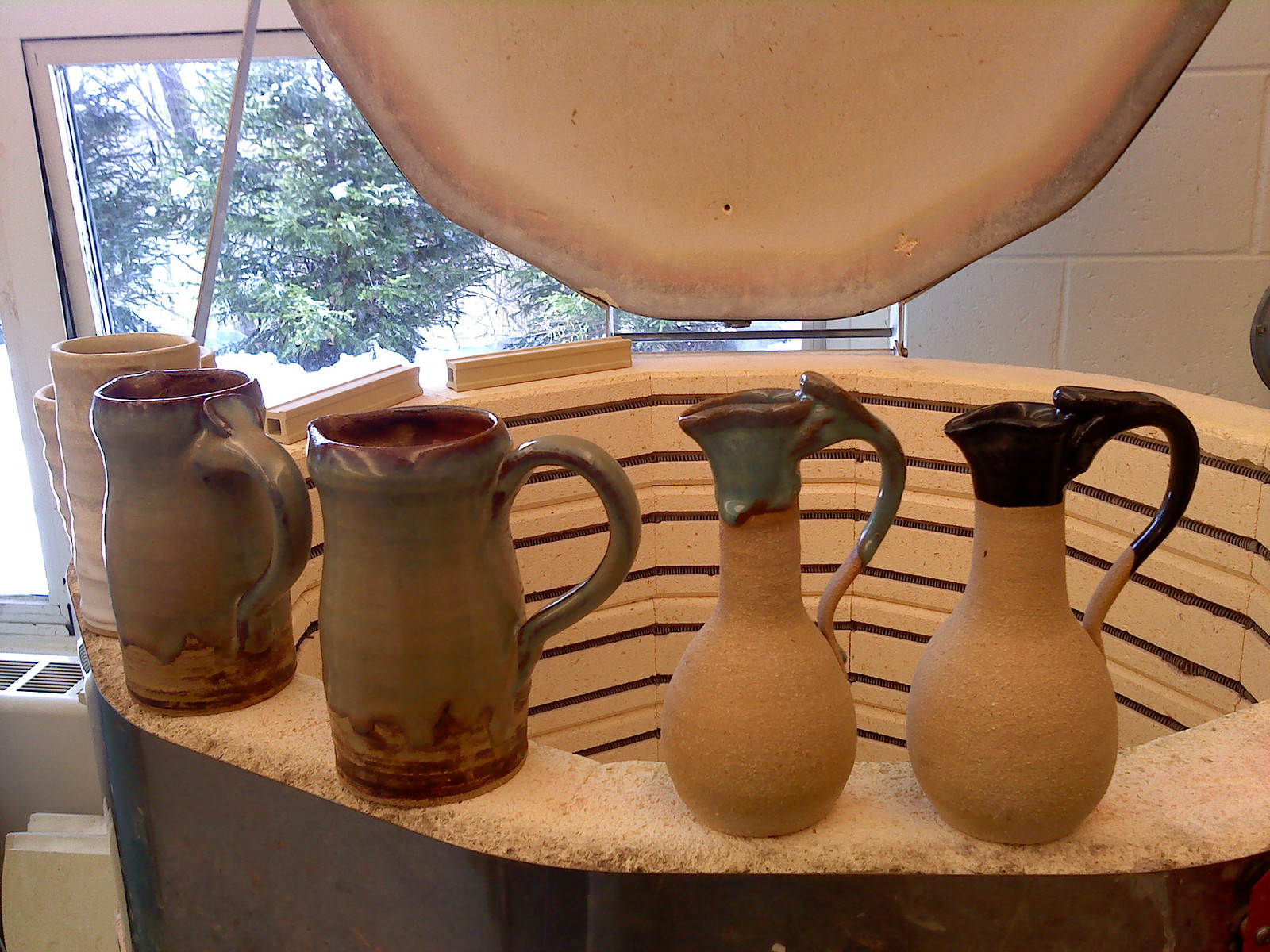The photograph captures an indoor scene centered around a prominent, cylindrical stone structure, resembling a hot tub or large basin, situated within a home. The structure, made of a white stone with visible horizontal stripes, features an open lid revealing its interior. Arranged atop this basin are a collection of pottery pieces, including six ceramic water pitchers in varying colors and designs. To the right, we see two ornate pitchers with green tops and beige bottoms, tapering at the base. On the left side sit two green pitchers alongside two white ones, all with rounded handles. The scene is framed by a large window streaming natural light and offering a view of dense greenery outside. Suspended above the basin, partially visible, is a white stone disk, adding a touch of elegance to the setting.